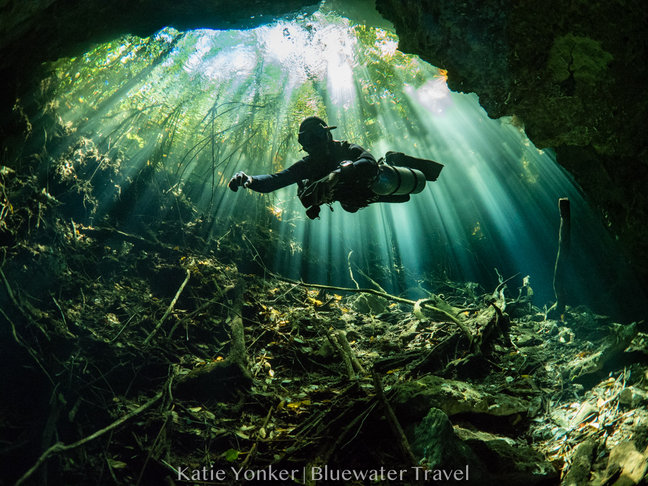In this captivating underwater photograph, a scuba diver is captured exploring what appears to be an underwater cave. The diver, positioned in the middle of the image and silhouetted by sunbeams streaming down from the surface, is equipped with a mask, a large air tank, and flippers, and appears to be swimming towards the camera. The lighting from above highlights a scattering of natural debris, including tree branches and leaves, on the cave floor. Framing the scene, dark rock formations are visible both in the upper left and upper right corners, adding depth and a sense of adventure to the image. Beyond the water’s surface, faint outlines of trees or plants are discernible, hinting at the world above. At the very bottom of the image, the caption reads "Katie Yonker, Blue Water Travel."